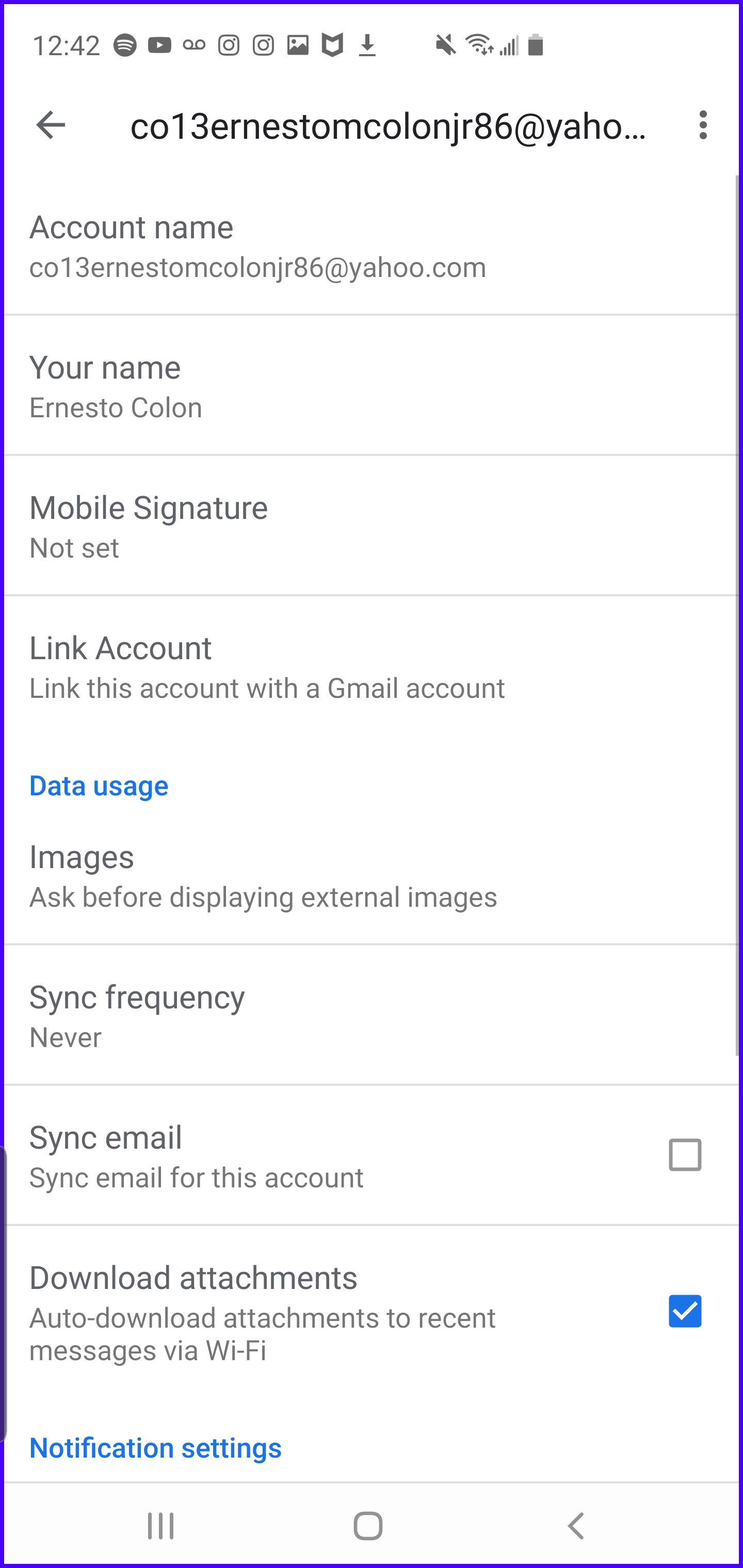A detailed image caption may look like this:

"A screen capture from an Android or Samsung smartphone displaying the account settings for a Yahoo email account. The top of the screen shows the account's name as 'Co13ErnestoMCologneJr86' with a truncated email address, visible only as 'Y-A-H-O...'. The account holder's name, Ernesto Cologne, is shown prominently below. The screen indicates that a mobile signature is set, and an option to link this account with a Gmail account is presented. The next section, highlighted in light blue and labeled 'Data Usage,' lists various settings: The 'Ask before displaying external images' option is enabled, the sync frequency is set to 'never,' the 'Sync email' option is unchecked, but the 'Download attachments' option is checked, allowing automatic download of attachments from recent messages when connected to Wi-Fi. The section ends as it begins another light blue header for 'Notifications,' which is partially cut off and not visible in the screen capture."